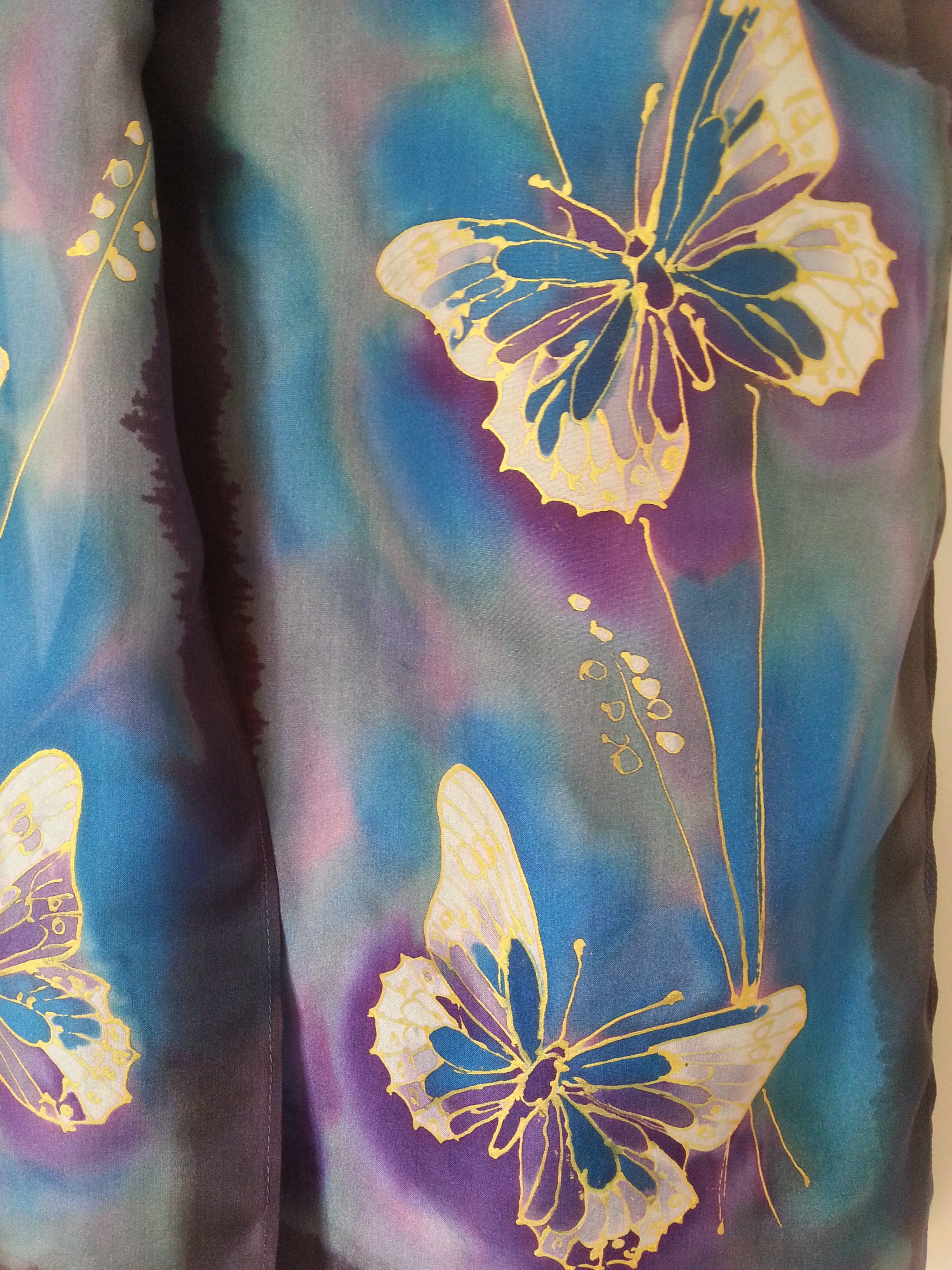The image features a detailed watercolor painting of butterflies set against a multicolored background composed of soft hues of blue, pink, yellow, and black, creating a dreamy, ethereal effect. The background has a faded watercolor wash, mixing light gray-green, pink, mostly purple, and some darker blues in a kaleidoscope-like pattern. In the foreground, there are two fully visible butterflies and part of a third butterfly’s wings on the left side of the image.

Both fully visible butterflies are located on the right side: one at the top right and one at the bottom right. The butterflies are adorned with striking colors that mirror the background, including yellow, blue, and purple. The wings feature gold edging and blue and purple interiors, with the centers and tails tinged in a deep purple hue. They are also characterized by having two slender antennae each.

Interwoven with the butterflies, delicate gold lines mimic the appearance of twigs, with tiny yellow leaves or small filled flowers attached, adding a botanical element to the scene. The overall effect is a harmonious blend of nature-inspired elements and vibrant, fluid colors, creating a visually captivating and intricate composition.